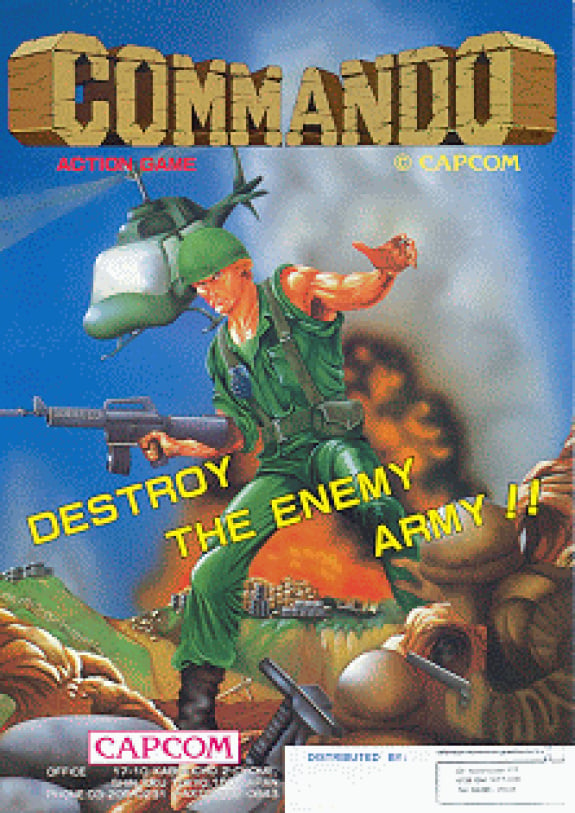This is a vertical, rectangular image of the cover of the video game "Commando." In the center of the image stands a soldier dressed in a green uniform, equipped with various gear and a belt. His right hand clutches an automatic rifle, possibly an AK-47, while his left hand is outstretched, appearing to maintain his balance on uneven terrain. Directly behind the soldier is a massive plume of smoke arising from an explosion, adding a dramatic backdrop against the solid blue sky. The explosion seems to originate from a distant city skyline. 

To the left of the soldier’s head, a helicopter hovers, enhancing the picture's intense, warlike atmosphere. In the foreground, several soldiers dressed in tan uniforms and army helmets emerge from a trench, facing the central soldier and appearing to engage in combat.

At the top of the image, the title "Commando" is prominently displayed in a semi-circle of golden, stone-carved letters. Below "Commando," the phrase "Action Game" is written in small red letters, and "Capcom" is positioned on the right side underneath the title. Across the lower half of the soldier, the text "Destroy the Enemy Army" appears in bold yellow letters. Additionally, the bottom left corner of the image features the "Capcom" logo, adding a final touch to this action-packed cover art.